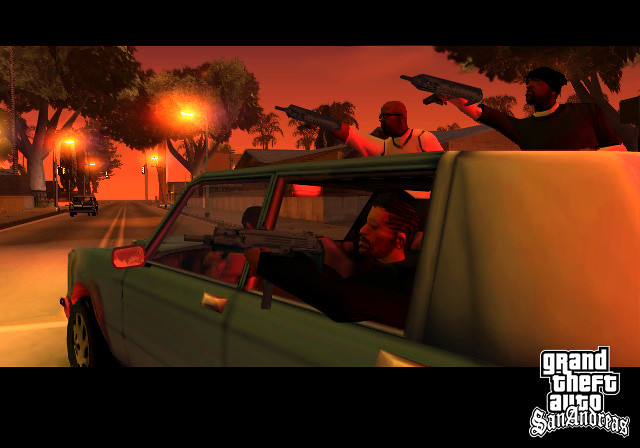Screenshot from the video game Grand Theft Auto: San Andreas: The bottom right corner features the game's iconic logo. Horizontally across the top and bottom edges of the image are black strips framing the scene. The focal point is an 80s-style green car occupied by four men, all appearing to be Black. The man in the front passenger seat wears glasses and a white shirt, while the man in the back left passenger seat sports dreadlocks. In the back right seat, a man with a black beanie and brown shirt is visible. Two additional men, brandishing guns, lean out from the front and rear passenger-side windows, aiming to the left. A white sheet covers the rear of the car. The scene is set on a residential street riddled with trees, captured at sunset, casting a dim light over the surroundings.